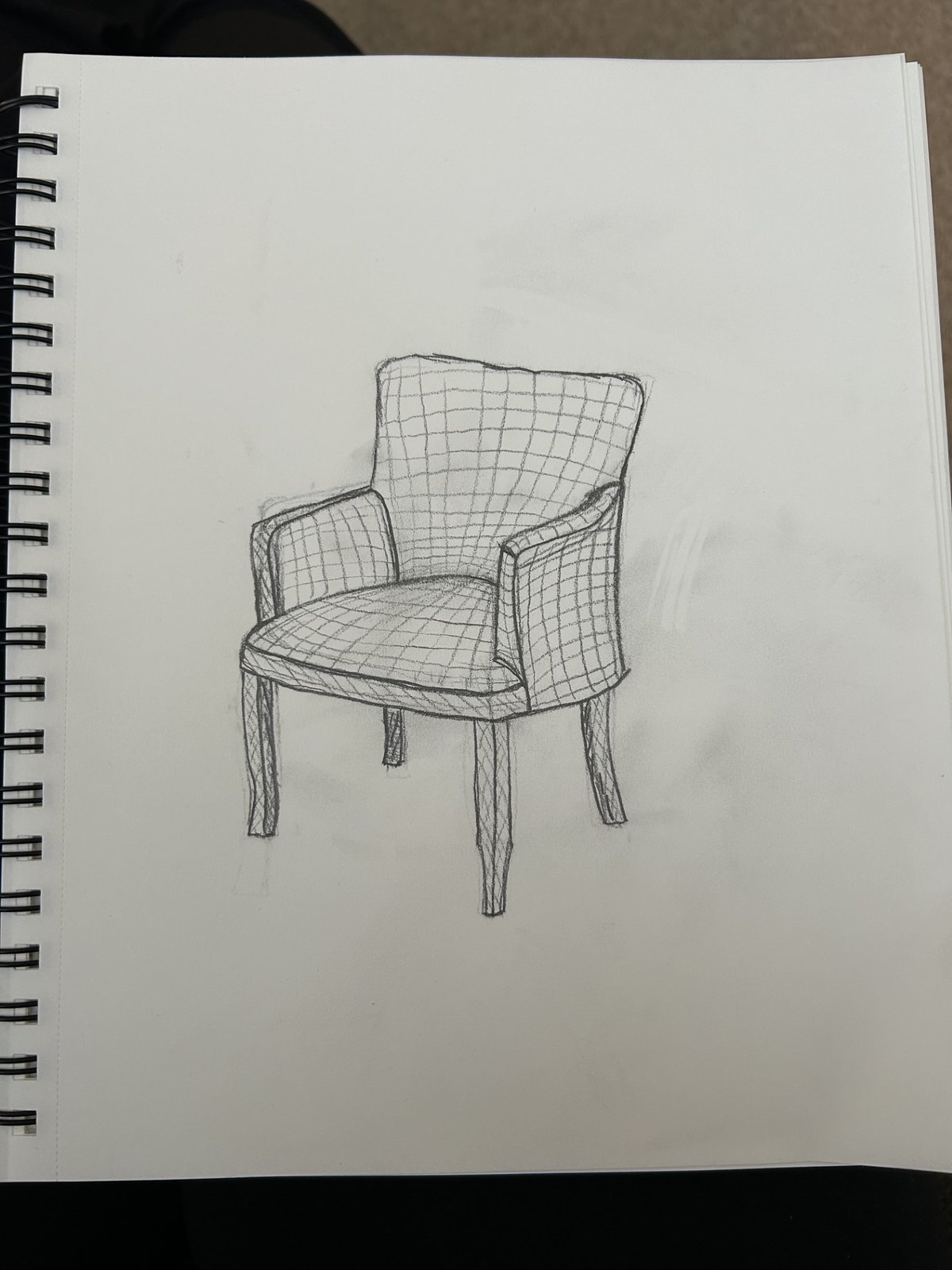This image features a detailed sketch of a chair, positioned diagonally to the left. The chair prominently displays four legs, with two legs visible on each side. Its cushion, armrest, and backrest are intricately sketched with a grid of horizontal and vertical lines, creating a pattern of small, square-like shapes that cover the entire surface of the chair. In the lower portion of the image, a rectangular black background adds a contrasting element, extending slightly upwards. On the left side of the sketch, a series of black rings can be observed, indicating the spiral binding of the white-paged notebook in which this detailed chair illustration has been crafted.